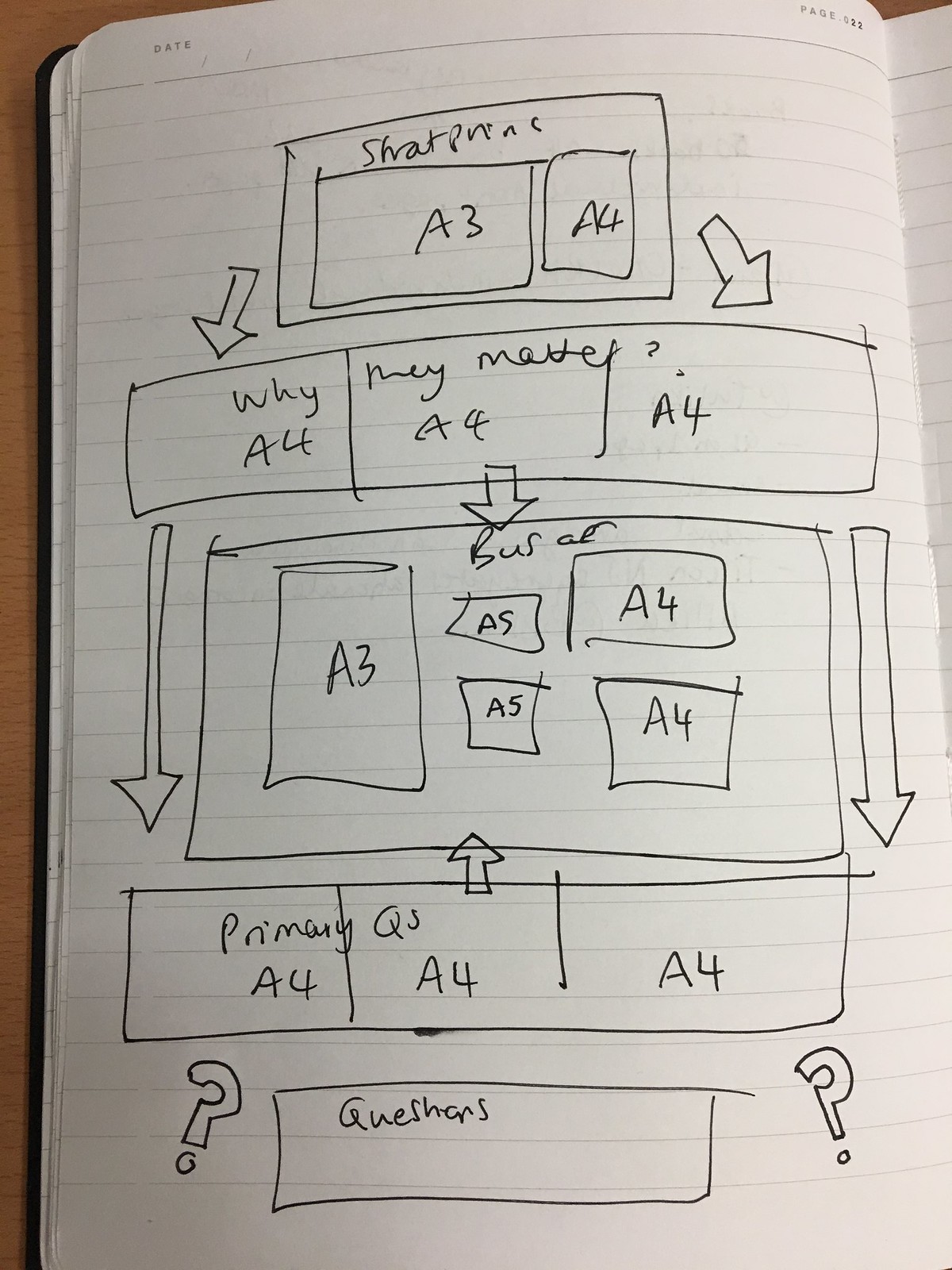This photograph captures a hastily drawn flowchart in someone's notebook, featuring white, lined pages. The diagram appears complex and difficult to interpret, likely intended solely for the creator's use. Details are hard to discern, as the handwriting is particularly rushed.

At the very top of the flowchart, a large rectangle contains two smaller rectangles: one rectangular and labeled "A3," the other more square and labeled "A4." A somewhat illegible word, possibly "sharpness," is written above this, but cannot be confirmed.

From this top rectangle, two arrows descend on either side, pointing to a wide rectangle labeled with multiple entries: "Y," "A4," "my money," "A4," and "A4." Following this, another arrow extends downward, connecting to a rectangle compartmentalized into five smaller rectangles, labeled "A3," "A5" (two instances), and "A4" (two instances).

Continuing downward, the next rectangle is connected by arrows from the edges of the previous rectangle. This section is labeled "primary cues" and includes "A4," "A4," and "A4." A small arrow loops from this rectangle back up to the rectangle above it.

At the very bottom lies a rectangle labeled "questions," flanked by question marks on either side. The entire diagram is sketched in black pen, highlighting an intricate but somewhat chaotic thought process.